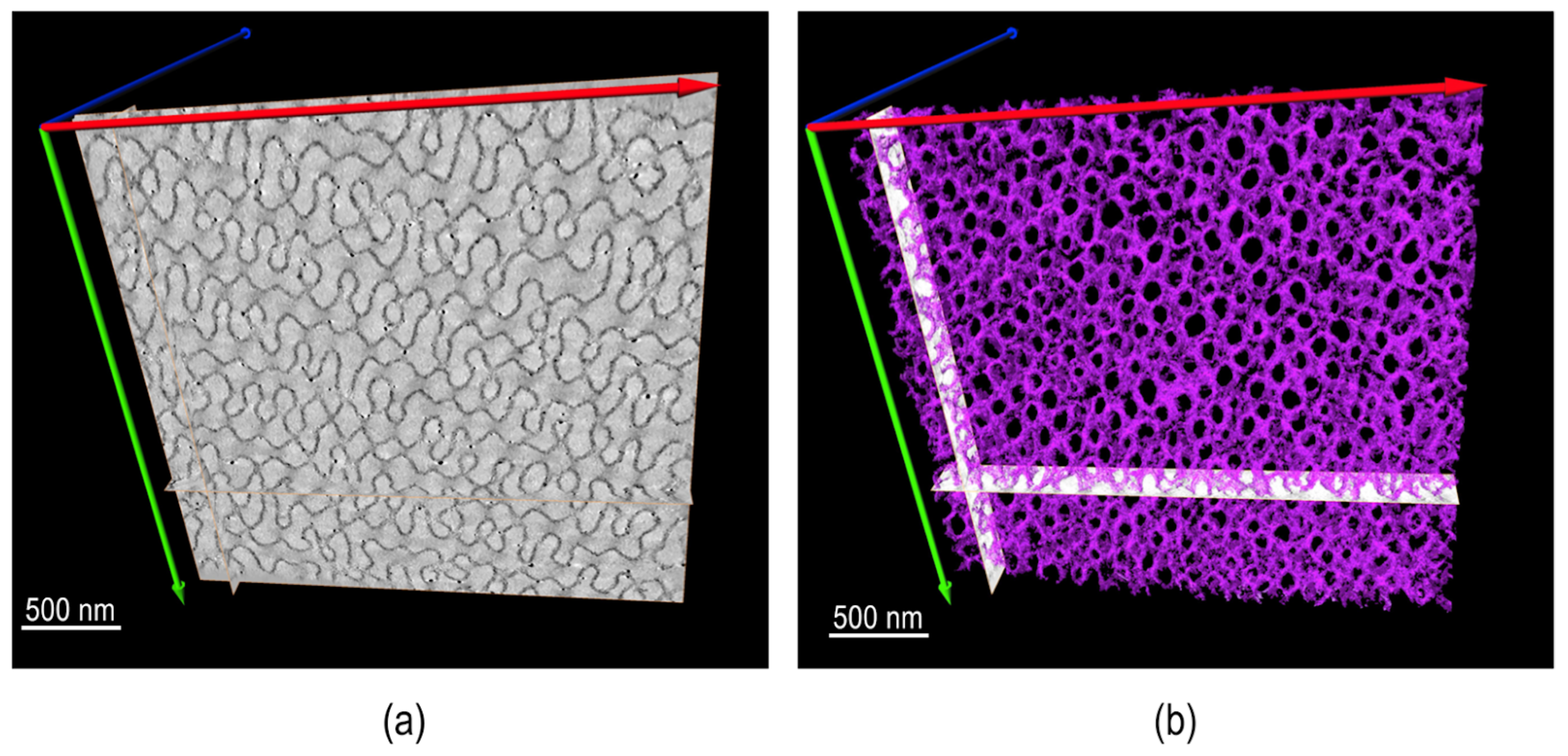The image consists of two computer-generated graphics, labeled "A" and "B," set against black backgrounds. Each section features a square, with both squares being marked "500 nm" in the bottom left corner, indicating their size in nanometers.

In Section A, the square is gray with a pattern of darker gray squiggly lines. Three colored arrows are present: a red horizontal arrow indicating length, a blue arrow pointing backward suggesting depth, and a green vertical arrow indicating height. These arrows outline the dimensions and orientation of the square, resembling the depiction of a 3D object.

In Section B, a similar square appears, but it is purple with fluorescent properties. The colored arrows—red, blue, and green—are arranged in the same orientation as in Section A. Additionally, this square is transparent, and two intersecting white lines form what looks like an X and Y axis, highlighting the square’s position more precisely. The contrast between the gray and purple squares suggests that the purple version might be displaying the material or object under special lighting conditions, possibly fluorescence.